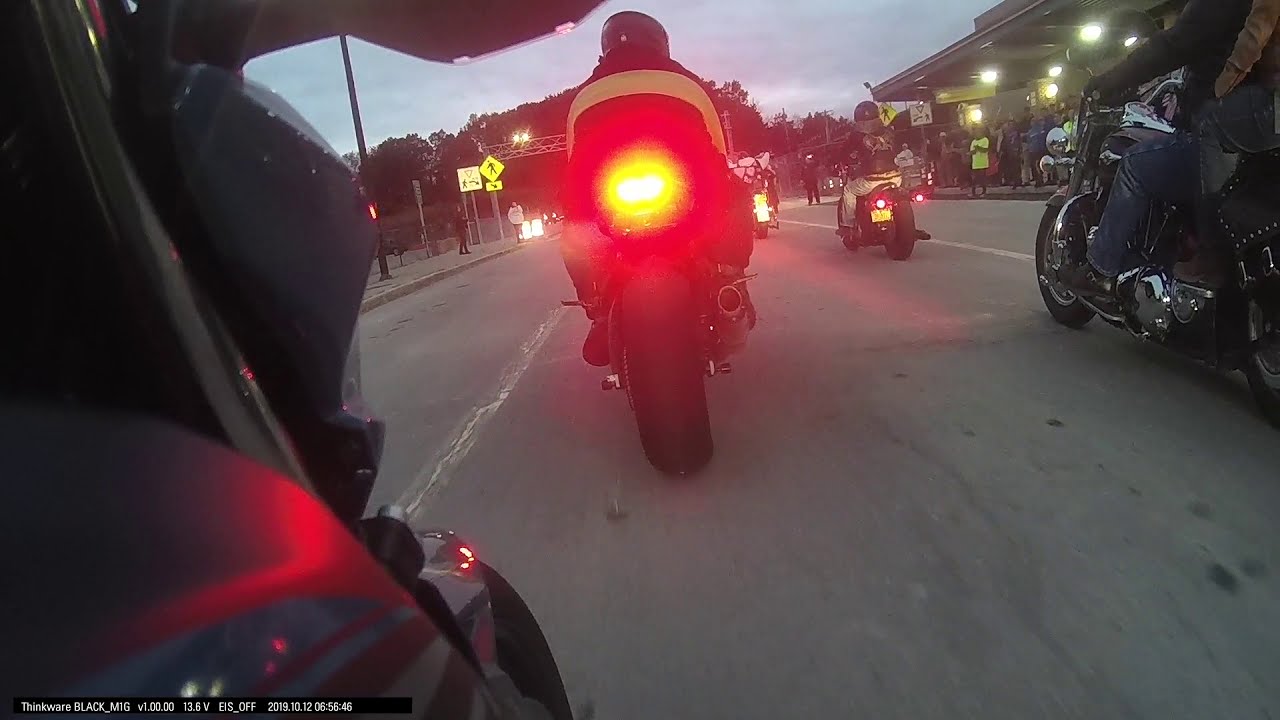The image captures a dynamic street scene centered around a group of motorcyclists, evidently moving forward. At the forefront, there's a motorcycle with a distinctive rear brake light, highlighted by concentric rings of white, yellow, and red illumination. To the left of the image, close to our viewpoint, another motorcycle appears prominently, suggesting a low-angle perspective, possibly from a camera attached to this bike. 

Further left, a sidewalk reveals additional motorcyclists, trees in the distant background, a telephone pole, and pedestrians. One person is clad in a black outfit, another in white. More motorcycles are visible to the right, aligned neatly next to each other. The pavement below appears aged, marked by cracks and oil stains, indicating a well-used road.

On the right side of the scene, buildings brighten the dusky sky with their lights, particularly those under an awning, where a crowd has gathered as if watching a parade. The spectators, dressed in various colors, lend a festive air to the scene. The sky above shows signs of evening with patches of gray, enhancing the prominence of street and building lights. The combined details suggest a lively, communal atmosphere amidst the motorcyclists and onlookers.